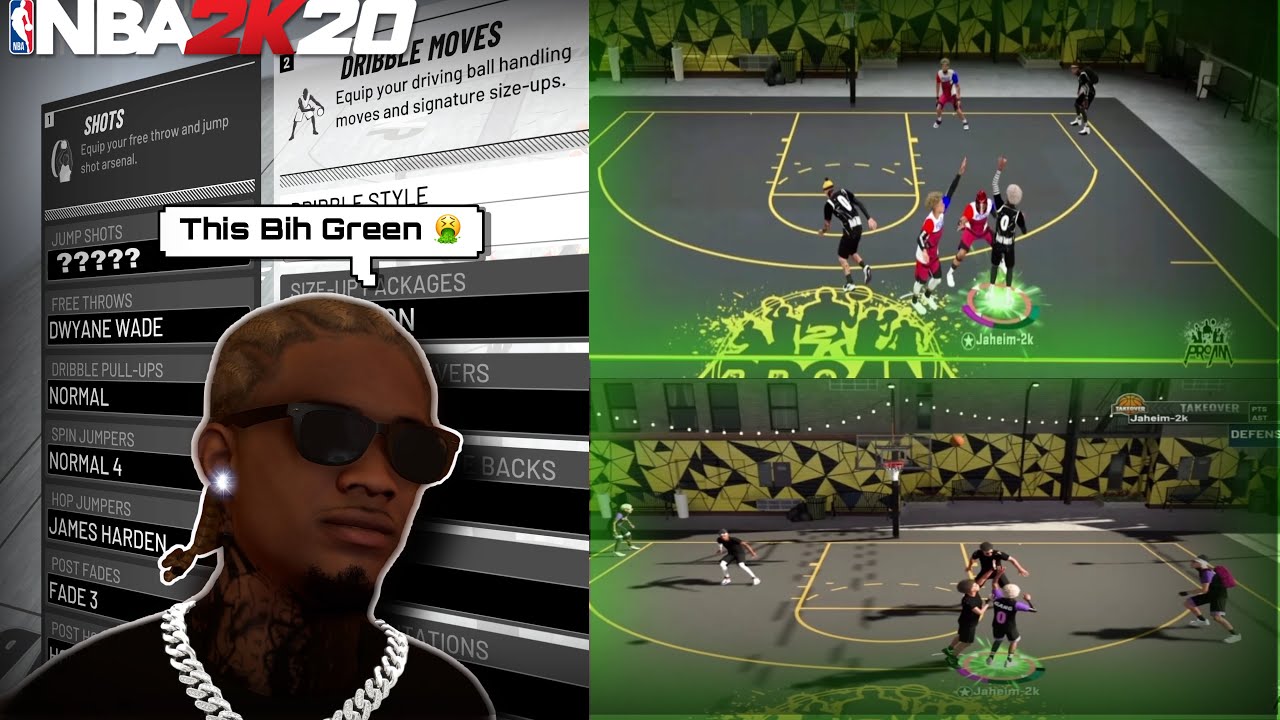This image appears to be from the video game NBA 2K20, as indicated by the prominent NBA logo in the upper left corner. The logo features a silhouette of a basketball player with a blue stripe behind him on the left and a red stripe behind him on the right, with "NBA" written in white at the bottom left. Below that, "NBA" is written in white, "2K" in red, and "20" in white, creating the game's title.

The screen is divided into two halves. On the left side, there is a close-up of an in-game character, a black man visible from the shoulders up. He is wearing black sunglasses, has cornrows, a black mustache, and a goatee. A large, silver chain hangs around his neck. Above his head, a speech bubble reads "this BIA green," accompanied by a vomiting emoji. Behind him, several instructional text boxes outline gameplay features: "Equip your free throw and jump shot arsenal," and "Equip your dribbling ball handling moves and signature size-ups."

On the right side, the image showcases a computerized basketball court within the game. The top part of this section shows an indoor stadium, while the bottom part displays a similar scene with players actively engaged in a basketball game. This vividly captures the dual aspects of player customization and in-game basketball action.